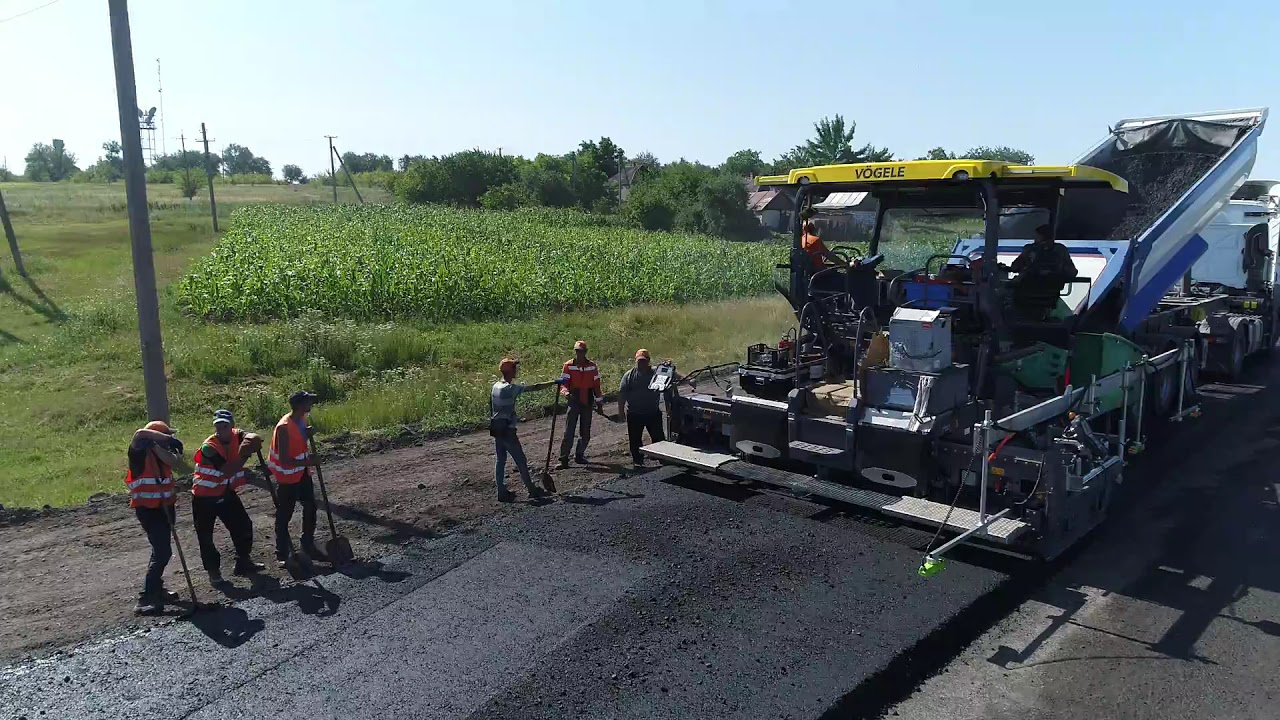The photograph, taken outdoors during the day, depicts a team of six workers dressed in orange vests and various headgear, including hats and helmets, working on a road surface. On the right side of the image, there is a large piece of construction equipment likely used for flattening or grading the road. This machine features steps and a long metal bar at the front and houses two seated operators managing controls. Behind this machinery is a truck with its back bed tilted upwards, pouring black gravel or asphalt into the machine.

In the foreground, freshly laid asphalt is visible, marked and smoothed over. The workers are seen leaning on shovels, waiting along the edge of the new pavement. Beyond the workers, a cornfield stretches out, interspersed with some tall vegetation and farm buildings. The background is completed with telephone poles and a mix of trees under a blue sky. The scene suggests a transformation of a former dirt road into a newly paved surface in a rural setting.